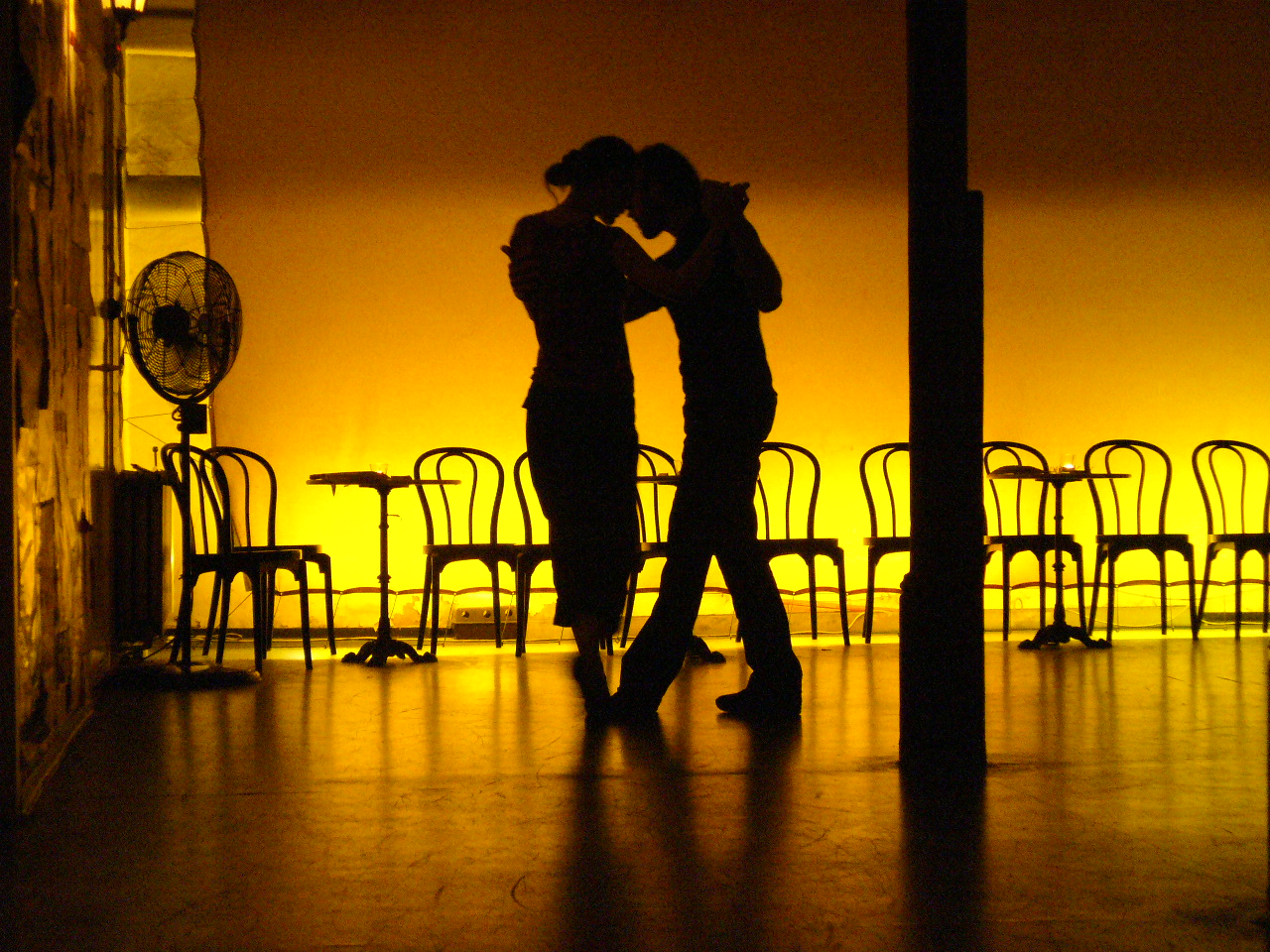In this warm, sepia-toned photograph, the focus is on the intimate silhouette of a man and a woman dancing closely together, their contours softened by the golden-yellow light that beams into the room. The woman, positioned on the left, has her hair pulled up into a bun and is donned in a flowing dress or skirt, while the man on the right is dressed in pants and a long-sleeved shirt. They are holding hands, their poses suggesting a romantic connection amidst the otherwise shadowy room. A large pole occupies much of the right side of the frame, offering a structural juxtaposition to the delicate moment shared by the dancers. Beneath them, a reflective concrete floor shimmers, enhancing the nostalgic ambiance. In the background, lined against the plain white wall, empty chairs hint at solitude or perhaps an event yet to commence. A stand fan in the corner subtly suggests a warm environment, a silent witness to the tender, private exchange captured just before sunset.